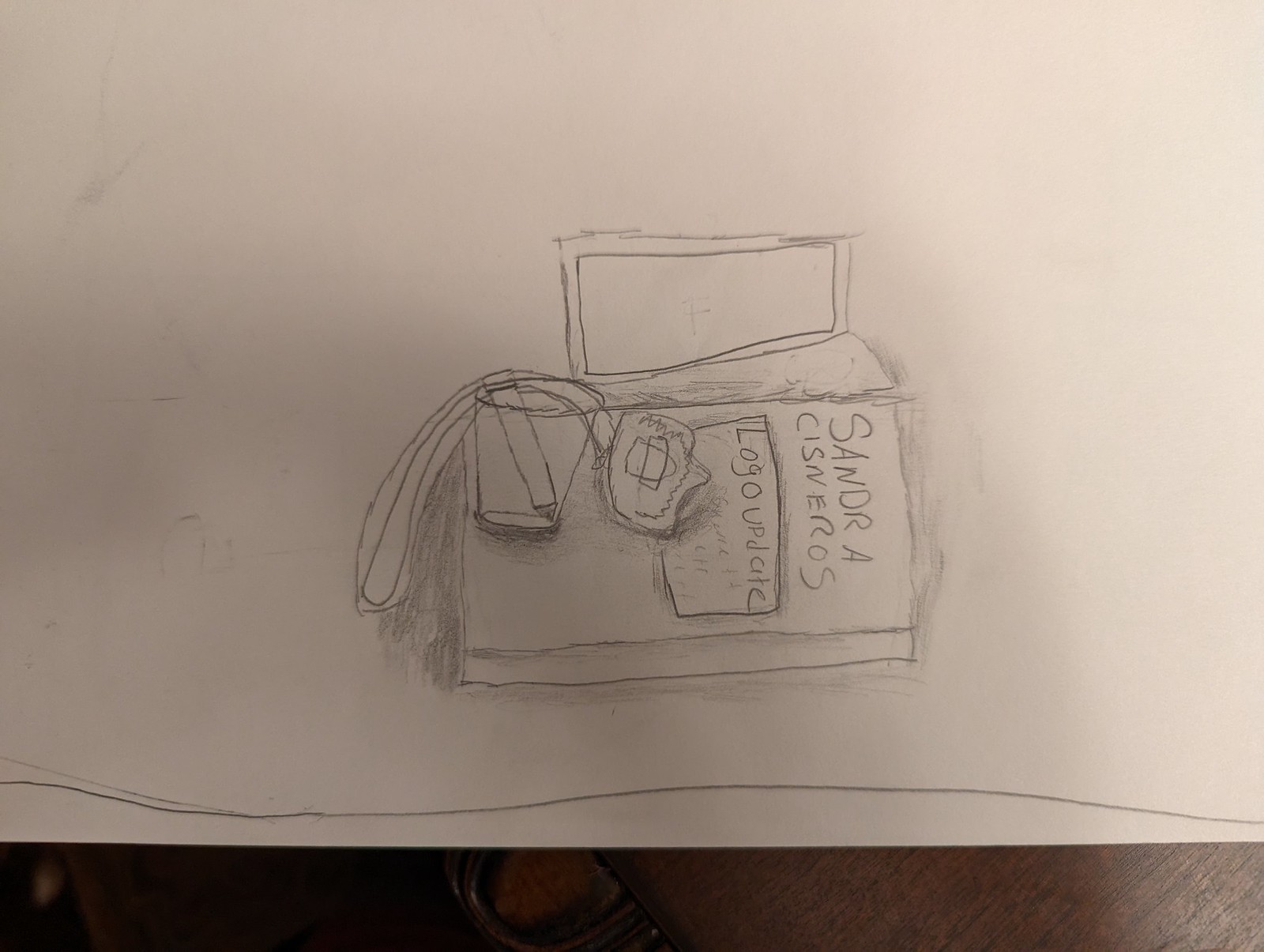A detailed pencil line drawing is sketched on a slightly off-white piece of paper, which rests on a dark brown wooden desk. The paper includes several pencil smudges, especially along its left edge. At the bottom of the paper, a thin wavy line runs horizontally. Central to the sketch is a square object that resembles a desk. On top of this "desk" is a rectangle with a border, suggesting a computer monitor. To the left, there's a basket-like container holding a pencil. Another rectangular box is positioned on its side in the center, bearing the words "Logo Update" at the top. On the right side of this box, the name "Sandra Cisneros" is written sideways. The drawing is simplistic but includes pencil shading and slight blurring to add texture and depth.